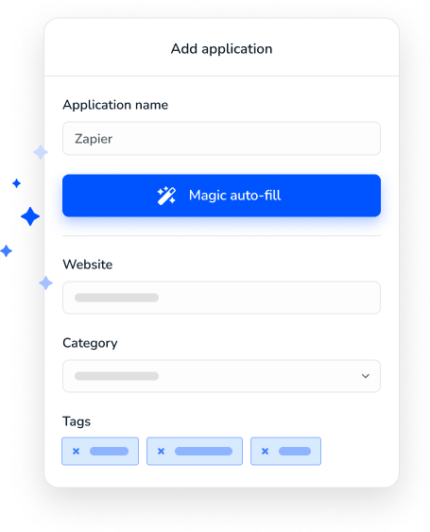This image depicts a portion of a larger user interface dedicated to adding an application. In this specific section, the application name "Zapier" is being entered, with the name clearly spelled out as Z-A-P-I-E-R. The interface also includes fields for inputting the website and category of the application. Users have the option to click a button labeled "Magic Auto Fill," which likely auto-populates some of these input fields, though the exact fields it affects are not specified.

Below these primary entry fields, there are designated areas for tags, allowing users to organize and categorize the application more efficiently. The layout seems designed to facilitate the creation of a website profile for the application, enabling users to input and arrange the necessary information in an easily findable manner.

Visually, the image is a fragment of a larger webpage, with no additional content visible outside this specific section. On the left side of the interface, there are decorative blue, four-pointed stars that add a subtle visual effect to the design.